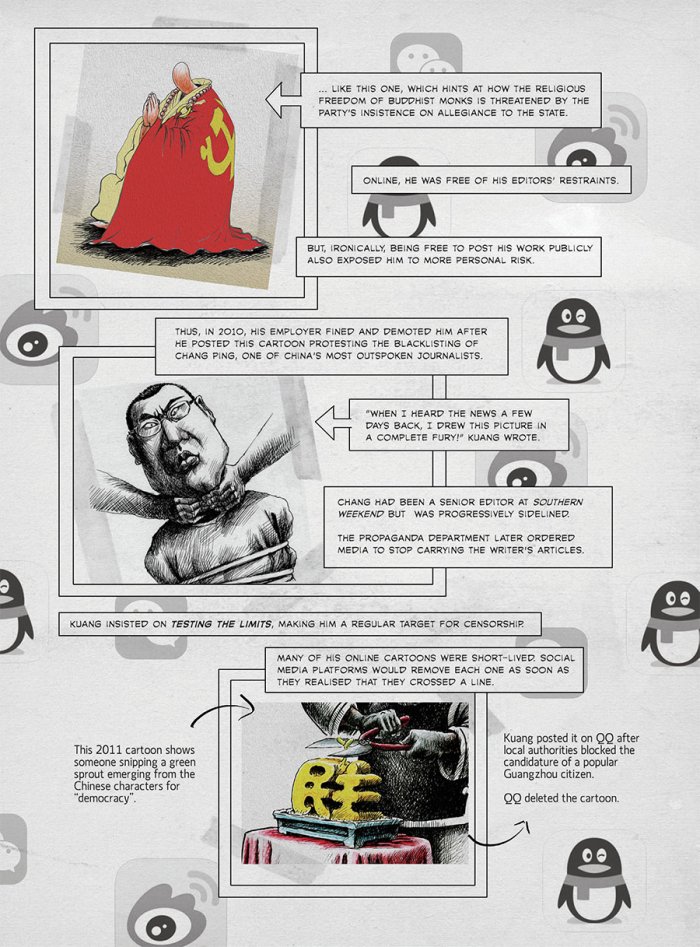This intricate illustration delves into themes of religious dissent and freedom of speech. Centered against a gray and white patterned backdrop is a human eye framed by a square, symbolizing scrutiny and surveillance. A playful penguin, winking and donning a scarf, adds an element of contrast. Scattered throughout the scene are black text bubbles, coupled with various elements of imagery. Notably, a prominent red religious figure is depicted wearing ornate red robes adorned with gold accents, both on the front and as a backdrop. Opposite this figure, a larger man with glasses is bound and being strangled, portraying oppression. In the concluding segment of the illustration, an individual is poised with garden shears, ready to cut a symbolic gold emblem, signifying the attempt to silence or alter religious expression. The entire piece critically addresses the plight of a journalist who faced repercussions from local authorities for creating a provocative, religion-themed illustration.